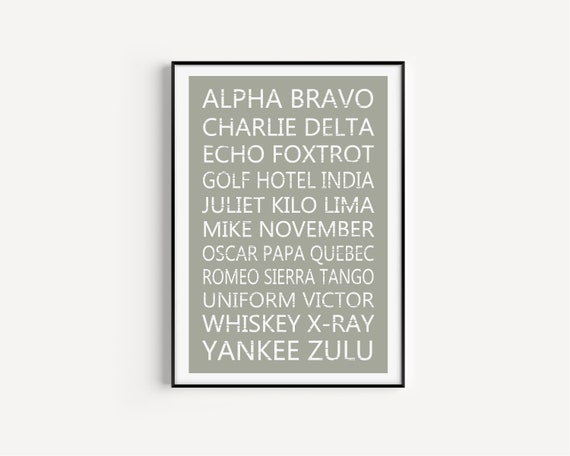This photograph captures a framed artwork displayed on a white wall. The artwork features a muted olive-grey background with white, uppercase text detailing the NATO phonetic alphabet used for clear communication of letter names. From top to bottom, the text lists: Alpha, Bravo, Charlie, Delta, Echo, Foxtrot, Golf, Hotel, India, Juliet, Kilo, Lima, Mike, November, Oscar, Papa, Quebec, Romeo, Sierra, Tango, Uniform, Victor, Whiskey, X-ray, Yankee, Zulu. The print is presented in a sleek, very thin black frame with a white mat border surrounding the text. The font has a somewhat retro feel, with some words appearing smaller to ensure everything fits uniformly within the framed space.